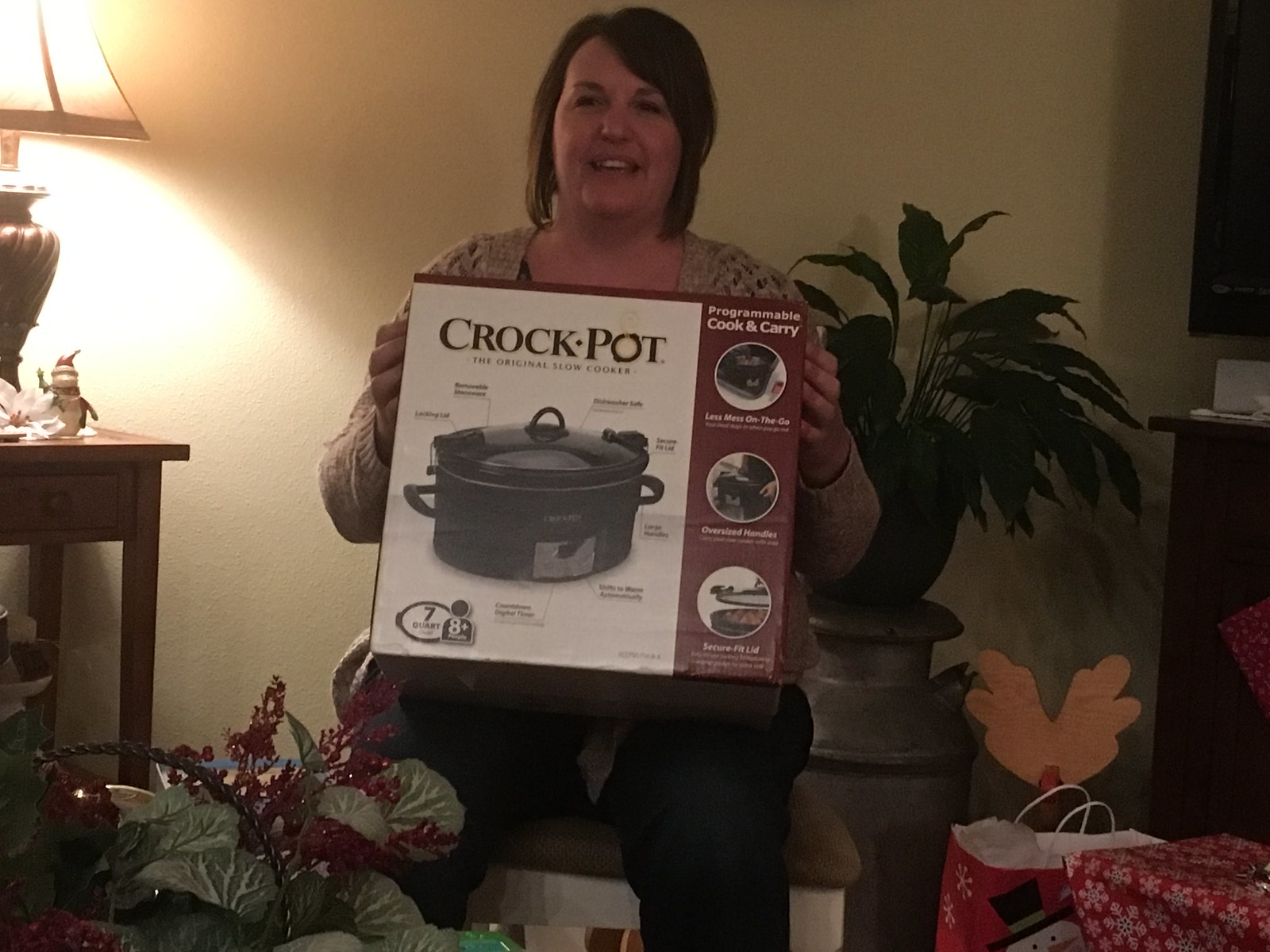The image captures a joyous scene of a woman sitting in a chair, holding an unopened box of a crock pot in her lap. She is presenting the box, which is white with a picture of a black crock pot and red font reading "Crock Pot," towards the viewer. The background of the box features three red circles detailing the crock pot's features. The woman is dressed in blue jeans and a light brown knitted cardigan, and she has short, shoulder-length hair. She looks happy, likely because she received the crock pot as a Christmas present.

To her left, a wooden coffee table with a lit lamp, a few small figurines, and a decorative snowman ornament is visible. To the right, there's wrapping paper, a red shopping bag with a snowman wearing a hat on it, and a red gift box adorned with white snowflakes. In front of her, a green plant with red decorative balls is placed next to a floral decoration featuring a basket with fake plants and red sparkly leaves. In the background, a vase with a plant on top completes the festive, cozy indoor setting.